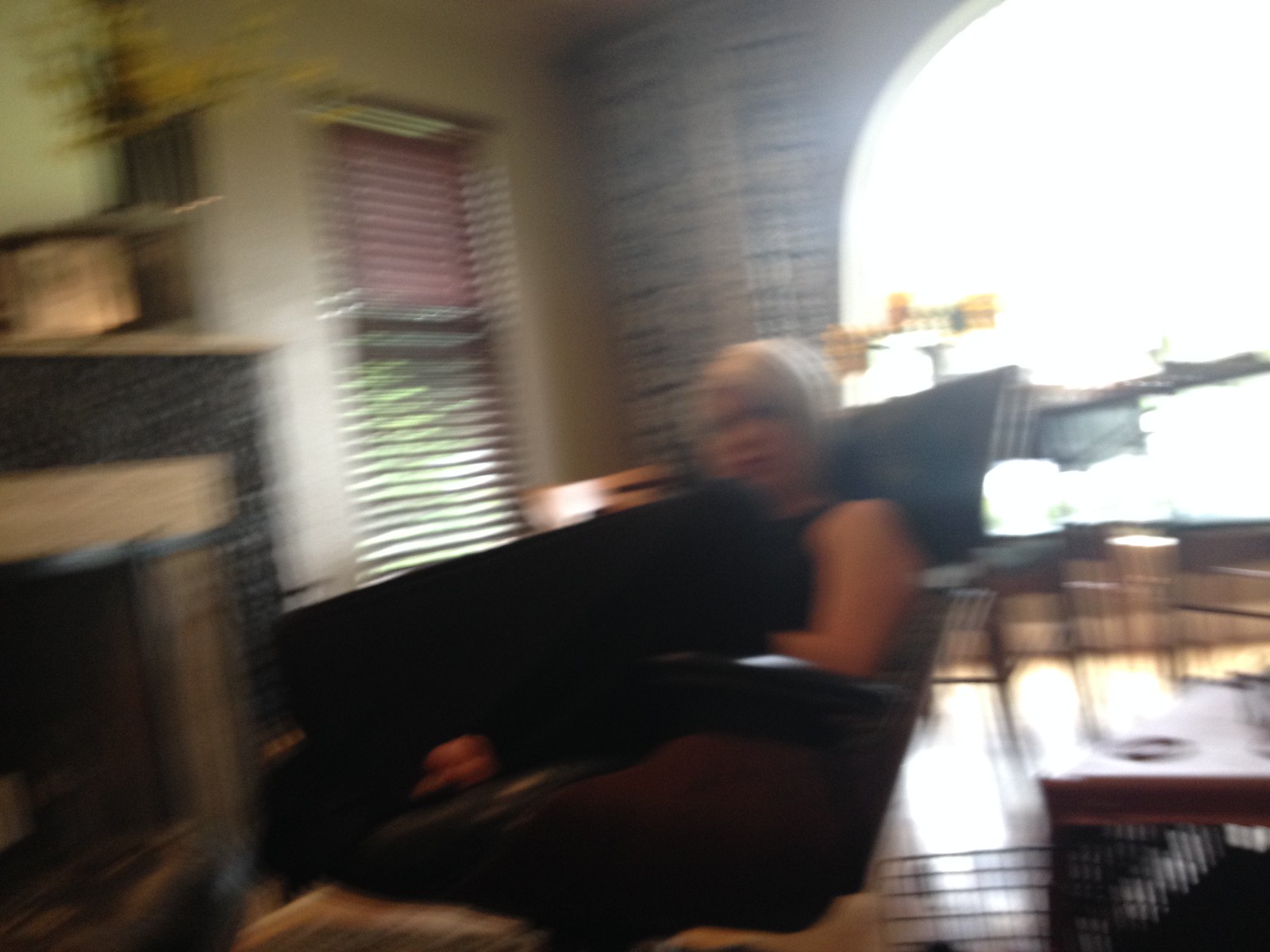This color photograph captures an indoor scene with a slight blur. At the center of the image is a woman seated on a beige plaid sofa. She is dressed in brown pants and a black tank top, with her blonde silvery hair cut just below her chin. She is wearing glasses and holding a long, black rectangular object in her hands. In the background, a beige stone fireplace with a darker mantel is visible. To the right, a window with open blinds allows natural light to filter in, revealing some greenery outside. An oval-shaped opening behind her further brightens the room with additional light. A table is positioned beside her, adding to the coziness of the setting.